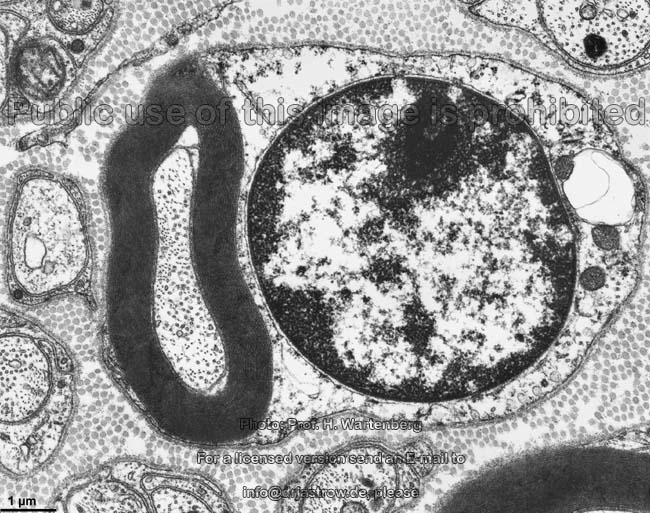This is a microscopic, black-and-white image capturing various microscopic organisms or cell types. The image is grainy and features numerous oblong and round shapes, each containing smaller shapes and specks. Dominating the center is a large black circle housing a white mass with many black specks. Surrounding this central feature, more faint gray specks scatter across the white background, and several smaller round and oblong shapes add complexity to the composition. Notably, a faint watermark stretches across the image, stating "public use of this image is prohibited." At the bottom, text reads: "Photo Professor H. Ortenburg. For a licensed version, send an email to info@drjastrow.de, please." Additionally, the bottom left corner indicates a measurement unit, likely "1 μm" (micrometer), enhancing the scientific context of the image.